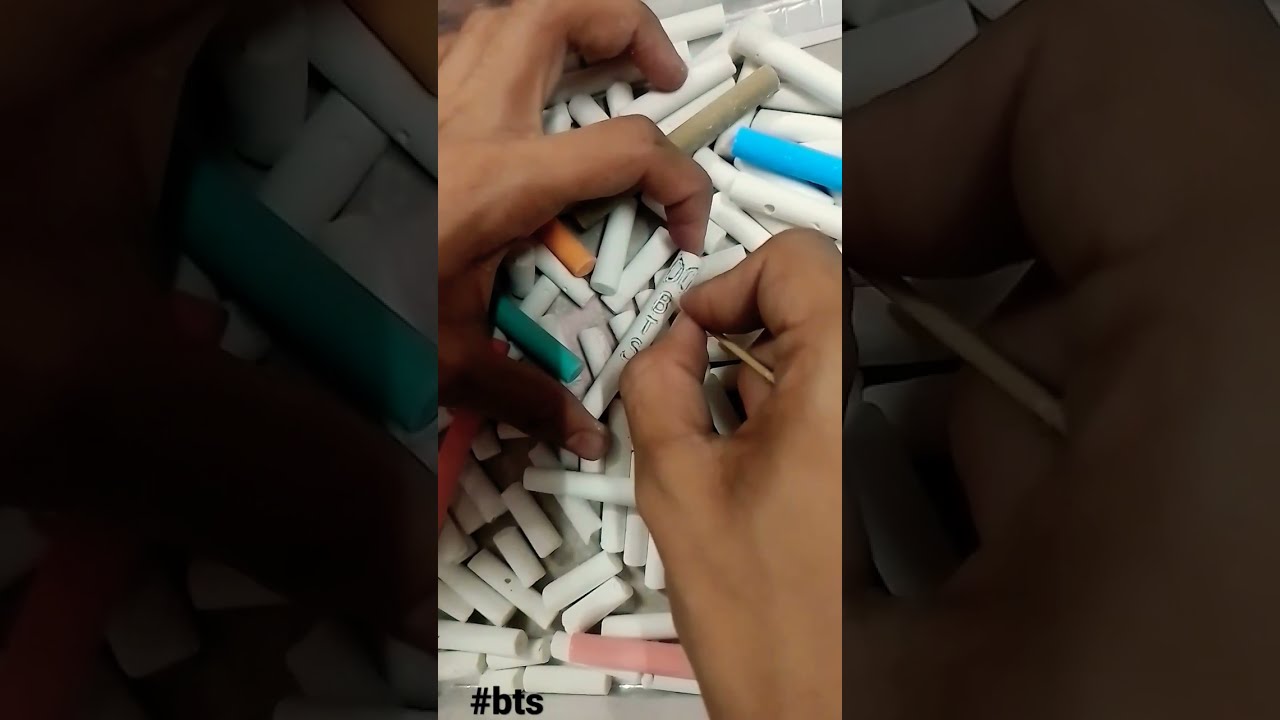The image showcases two light brown-skinned hands delicately engraving the letters "BTS" onto a white chalk-like stick using a toothpick. The hands' precise movements suggest careful attention to detail. Spread across the table are numerous short, smooth, straight sticks, predominantly white, but also featuring vibrant hues of blue, orange, green, pink, and brown. All the sticks appear to be made of a rubbery or plastic material. At the bottom of the image, there is a hashtag that reads "#BTS," connecting the artwork to the popular K-pop group BTS. The scene suggests an artistic project aimed at adorning each of these varied sticks with the BTS lettering.